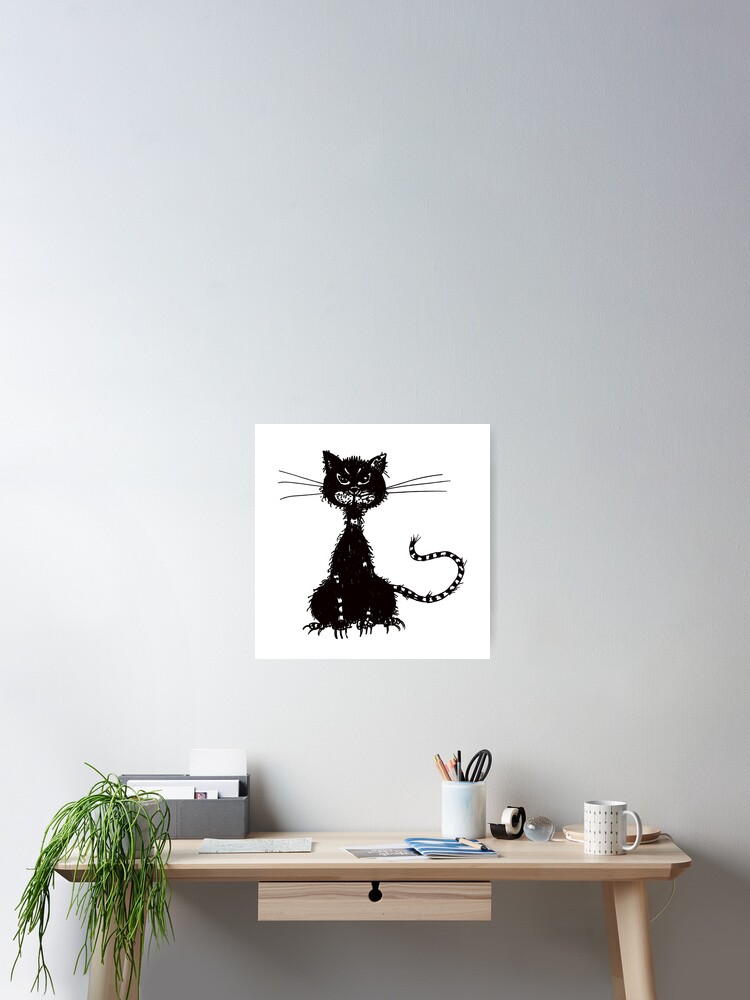The image depicts a minimalist setting with a wooden desk positioned against a plain white wall. Dominating the wall is a square picture featuring a black cat with menacing attributes—stringy, messy hair, oversized claws, pointy ears, and an unusually long, striped tail. The cat's expression is fierce, with long whiskers projecting a sense of anger or fear. Below this striking picture, the light brown desk supports various items, including a white lamp and a white coffee mug adorned with black dots, both on the right side. Centrally located on the desk is a tape dispenser alongside a cup holding scissors, pens, and pencils. Additionally, there is a small drawer integrated into the desk's design. On the left side, the desk houses a grey letter holder and a green plant with long leaves cascading over its edge. Scattered papers, including some blue sheets, and a book with a pen lie among the organized chaos on the desk's surface. The overall scene amalgamates simplicity and functionality, accentuated by the intense focal point of the snarling black cat artwork.